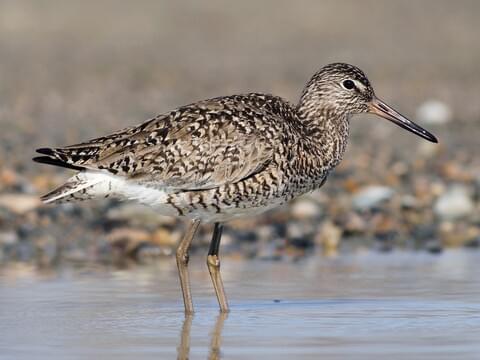This photograph captures an outdoor scene with a single bird standing in shallow, light brown water that reflects a hint of the blue sky. The bird has long, slender, tan-colored legs that bend backward at the knees, typical of bird anatomy. Its body is a mix of colors: a white underbelly becoming whiter towards the tail, adorned with brown and beige speckles and dark brown flecks. The tail features some black feathers while the overall body maintains a speckled appearance, providing a camouflage-like effect. The bird has a long, narrow bill that transitions from tan near the head to black at the tip, with visible nostrils. Notably, its eyes are black. The background is blurred, contributing to a foggy effect, and comprises an array of colored gravel including hues of tans, grays, blues, and darker shades. This setting appears to be a riverbank or the edge of a pond, devoid of any foliage, emphasizing the stark, natural environment.